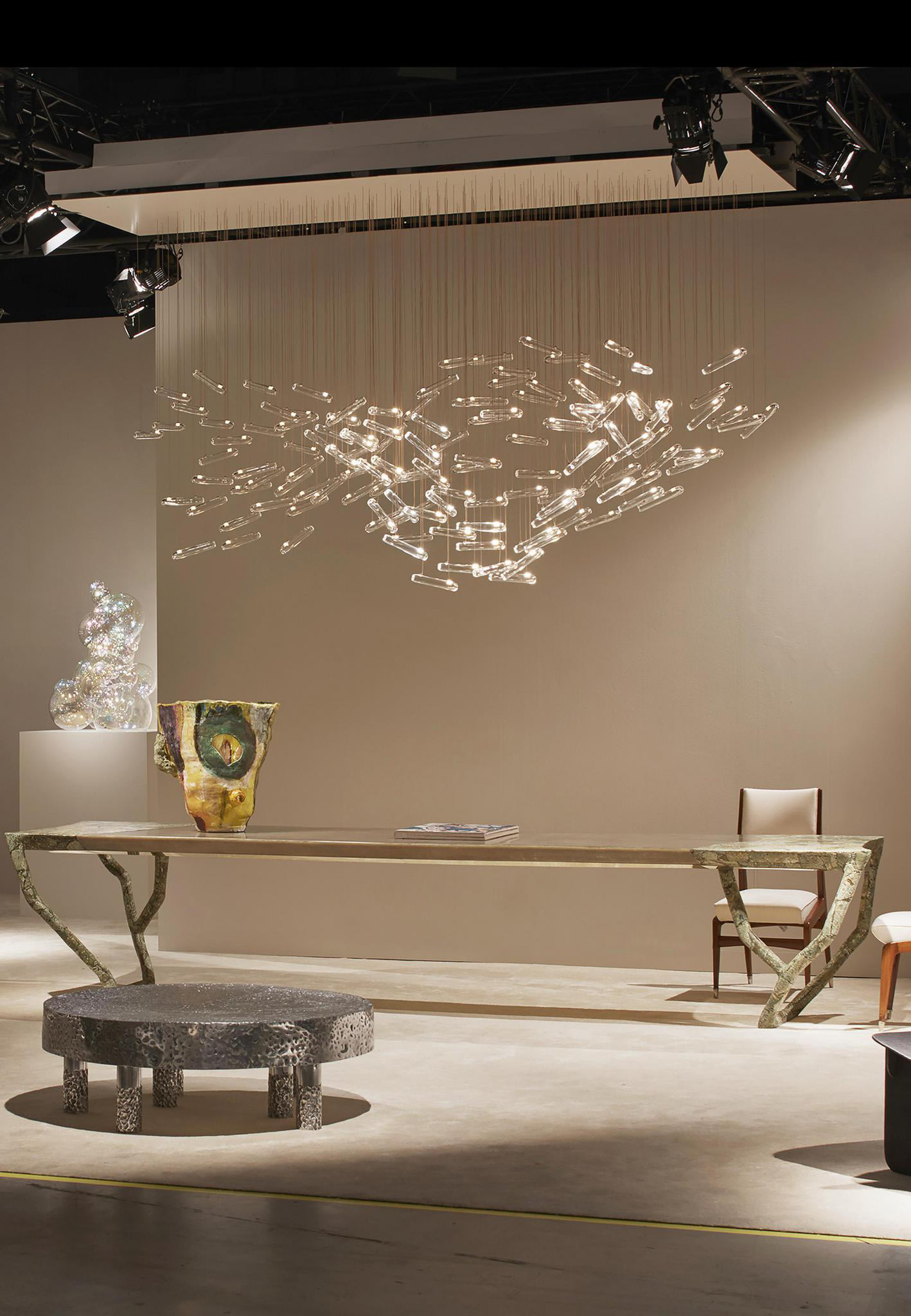The vertically rectangular, full-color photograph captures an intricately staged modern living room, elegantly lit with artificial lighting. The centerpiece of the room is a long table with legs resembling tree branches. Atop it rests a book and an eye-catching golden-green vase. Just behind the table, a single cream-colored chair is thoughtfully positioned. Hanging overhead is a distinctive lighting feature: a chandelier-like arrangement made from numerous thin wire hangers and clear crystal rods that create an intricate, fish-like pattern. This avant-garde chandelier is suspended from a beige rectangular ceiling fixture framed with dark brown trim, which houses projection lights in all four corners. The backdrop is a smooth beige wall, contributing to the room's refined atmosphere. In the lower left-hand corner, under the table, lies a round wooden stool, subtly lit from above, casting shadows across the cream-colored carpeted floor. Another similar stool can be seen in the far right corner. Adding to the artistic feel, a statue sits on a white pedestal to the far left. The room's unique blend of earthy wooden elements, modern art pieces, and sophisticated lighting gives it a contemporary, rich, and artsy ambiance.